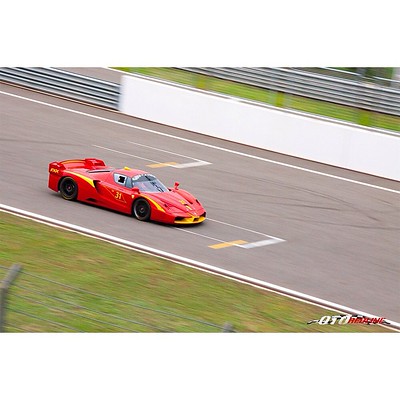This aerial photograph captures a bright tomato-red racing car in motion on a professional speedway track. The car, a sleek, low-to-the-ground sports model with black wheels and distinctive yellow accents, including yellow stripes on the hood and around the back wheel, is the only vehicle visible on the gray track. The track is bordered by white and yellow lines on both sides and features more of these markings behind the car. Blurry green turf flanks the track, indicating the car's high speed. There's a logo in the bottom right corner that reads "OTO," though the rest is illegible. The speedway is enclosed with a white guardrail transitioning to a gray one in the background. Additionally, a blurry indication of a small fence can be seen at the front, further emphasizing the car's rapid movement.